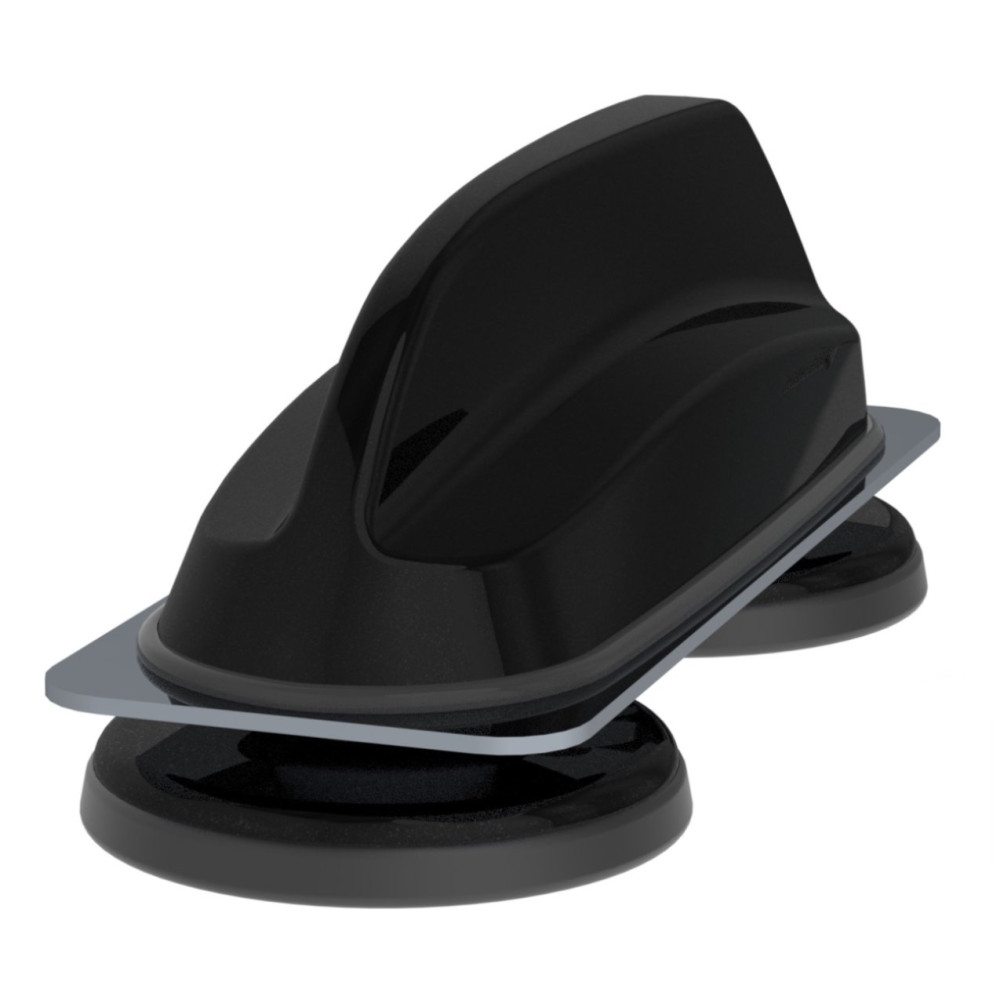The image depicts a close-up of a shiny, black, fin-style antenna typically seen on the back of cars or SUVs. The antenna's sleek, low-profile design resembles a shark fin, with smooth edges and a glossy finish. Below the fin, there is a flat black plastic base, which in turn, sits atop two circular pedestal-like structures. These circular structures, positioned with one in the foreground on the lower left and the other partially visible in the back right, resemble suction cups potentially used for mounting the antenna onto a vehicle. The entire setup rests against an all-white background, emphasizing its contrasting black and shiny surfaces.